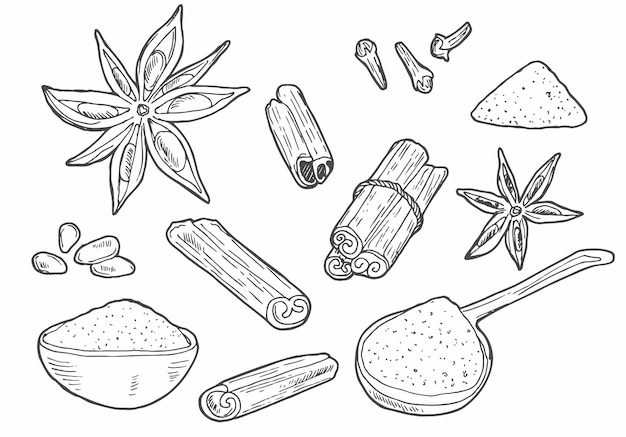This black-and-white sketch depicts a detailed assortment of various herbs and spices, artfully framed against a white background. At the core of the image, multiple cinnamon sticks are depicted, including a bundled trio tied with twine and several loose sticks scattered around. Prominently featured are two star anise pods, one smaller than the other, positioned near the cinnamon sticks. The top right corner showcases a small mound of powdered substance, likely a herb or spice, accompanied by three distinctive clove pods arranged in different directions: one angled down to the left, another slightly angled down to the right, and the last pointing up to the left. Additionally, a wooden spoon filled with powder and a small bowl containing another powdered seasoning add to the culinary tableau. Among these elements are what appear to be seeds, possibly pumpkin or sunflower seeds, enhancing the intricate composition of the sketch. This finely illustrated collection, potentially suitable for a textbook or cookbook, radiates a simple yet evocative representation of everyday kitchen spices, meticulously captured with pen and ink.